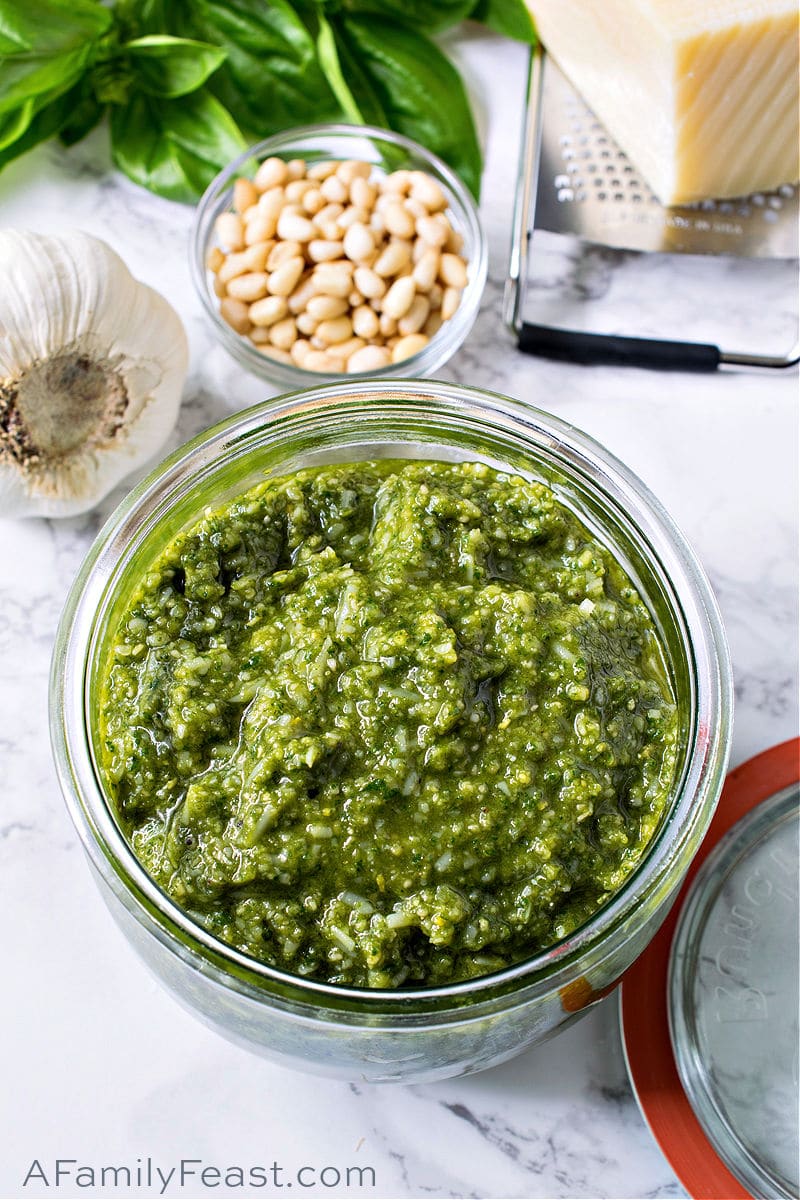This detailed photograph showcases a vibrant culinary scene atop a white marble countertop. The centerpiece is a large clear bowl filled with thick, vibrant green pesto sauce. Behind it, there is a smaller clear bowl containing what appear to be pine nuts. To the left of these two bowls lies a head of garlic. To the right of the pine nuts, there is a silver cheese grater with a block of white cheese resting on top. In the background, slightly to the left, fresh green basil leaves are arranged, suggesting that these are the ingredients for making pesto sauce. On the far right, there's the lid of a clear glass jar with a red ring around it. The composition suggests an inviting setup for preparing a delicious meal, with the website afamilyfeast.com noted at the bottom left corner of the image.